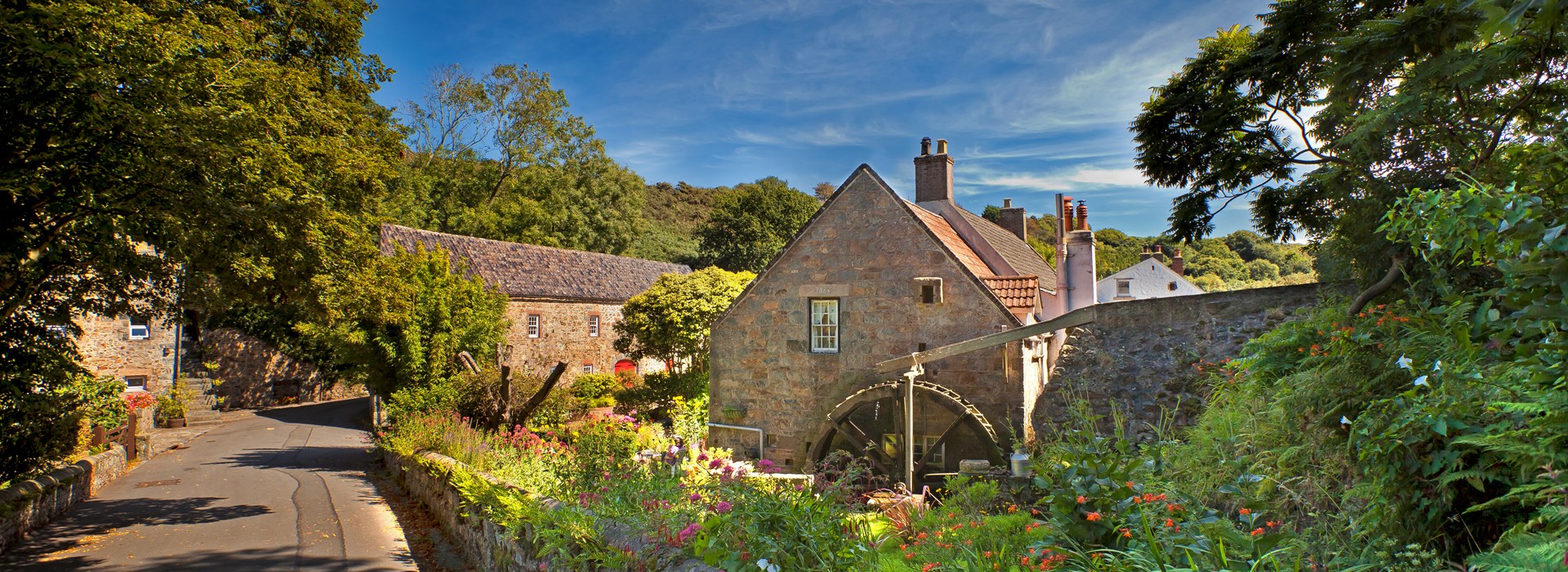The image depicts a charming rural scene that resembles a quaint European village, possibly English or Italian. The foreground showcases a winding asphalt path on the left, lined with lush pink flowers and green plants. Adjacent to the path, on the right, stands a quaint brown house featuring a triangular roof, two chimneys, and a prominent side window. Notably, a watermill is situated beside this house, hinting at a nearby canal. The left side of the image is adorned with large trees, while a row of red brick houses stretches out, resembling old warehouses with their robust yet charming appearance. In the backdrop, a majestic mountain rises against a brilliant blue sky dotted with fluffy white clouds. This idyllic, sunny landscape with its enchanting blend of natural beauty and historic architecture evokes a sense of timeless tranquility, as if it's a modern-day hobbit settlement.